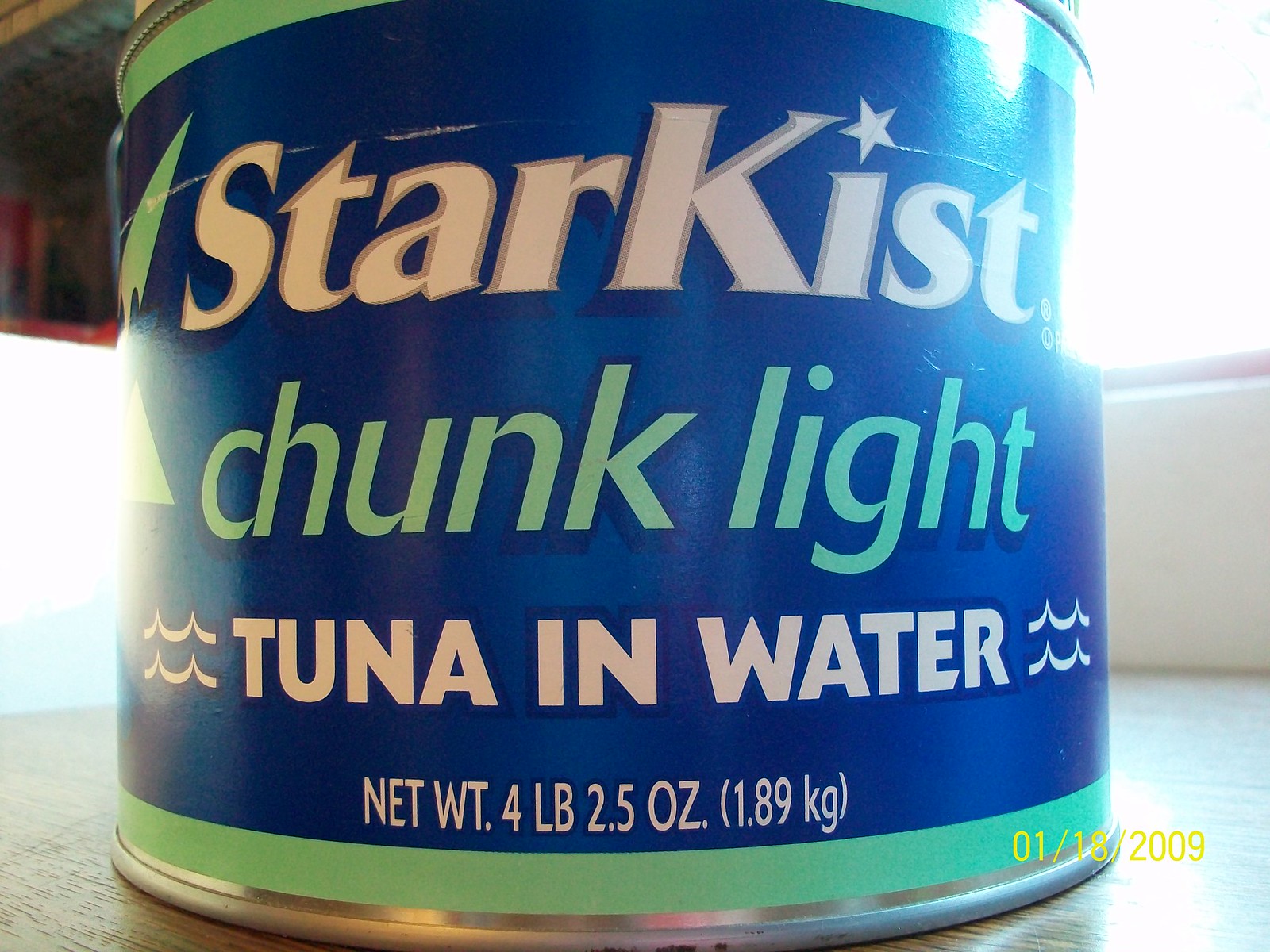This is a color photograph capturing a close-up view of a tuna can, occupying the full height and nearly the entire width of the frame. The bottom right corner of the image displays a yellow superimposed date, decipherable as "01/2009," though part of it is obscured by the can's edge. The background features a lighter patch emanating from a window on the right side, and a greyish wall. The can is placed on a wooden surface with a noticeable glare on the right. The left side displays a brownish hue. In the upper left corner, a brownish-grey roof edge is slightly visible.

The tuna can itself has a green rim at the top and bottom, sandwiching a blue background marked with white text and wavy lines. The top label reads "StarKist" in white, followed by "Chunk Light" in blue, and underneath, "Tuna in Water" flanked by wavy lines. Below this, the can's weight is indicated: "Net Weight 4 pounds 2.5 ounces (1.89 kilograms)." The detailed label and design elements suggest a well-recognized brand.